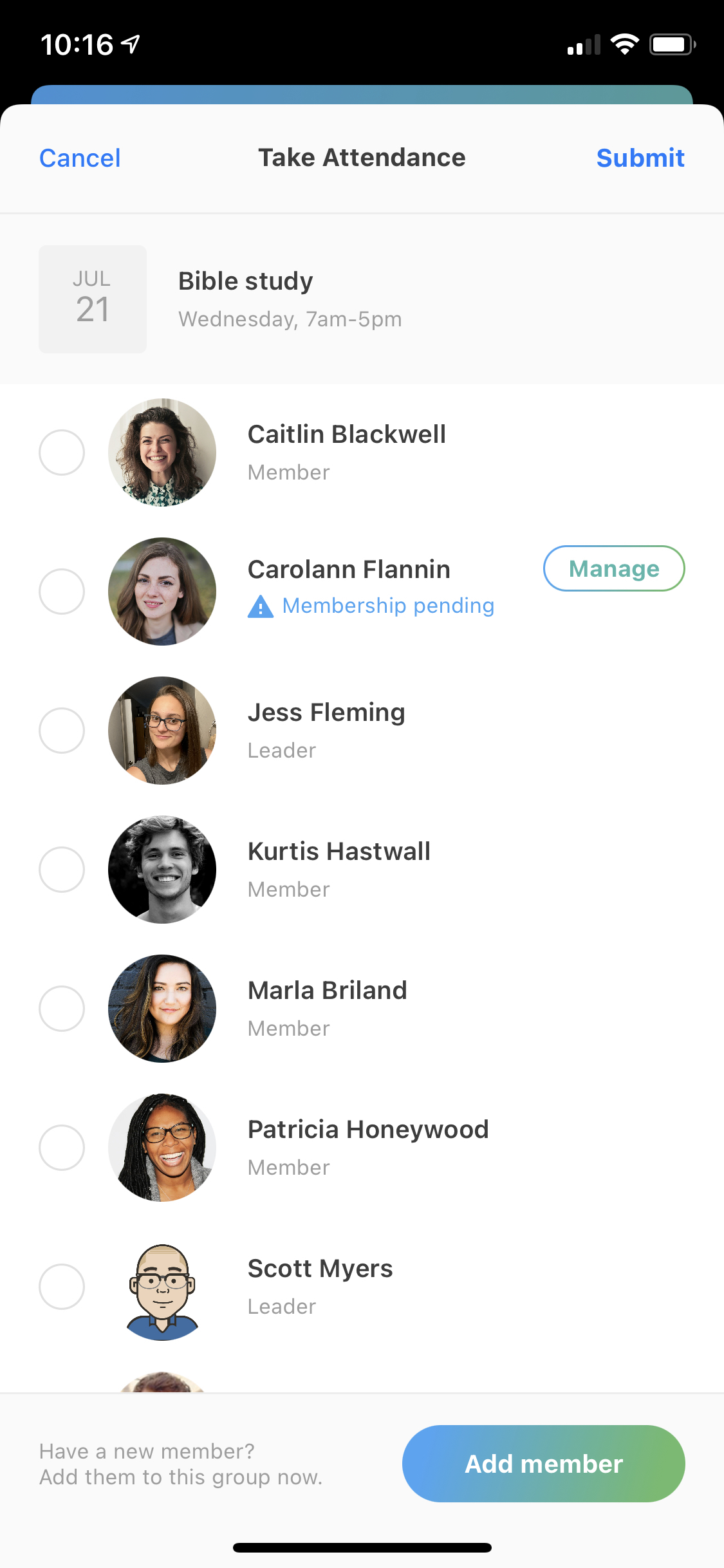This is a detailed screenshot from a mobile phone. 

At the very top, there is a black status bar displaying the time as 10:16 with white font. Additionally, it shows that location sharing is on. The mobile signal strength is indicated as two out of four bars, Wi-Fi is fully connected, and the battery is fully charged. 

Below this, there is an open menu displayed on a white background, which appears to be part of an app for a club or organization. The menu features blue font and is divided into several sections. At the top left, there is an option to 'Cancel'. In the center, the menu title 'Take Attendance' is highlighted. On the top right, there is a 'Submit' option.

The date "July 21st" is shown below this header, alongside the event description "Bible Study Wednesday 7 a.m. to 5 p.m.," indicating a long session duration. 

Further down, the app lists the members attending this event:

1. **Caitlin Blackwell** - Member
2. **Caroline Flannan** - Membership Pending
3. **Jess Fleming** - Leader
4. **Curtis Hastwell** - Member
5. **Marwa Breland** - Member
6. **Patricia Honeywood** - Member
7. **Scott Myers** - Member

Each member's status is displayed in small gray font beneath their names, giving a clear overview of their roles and membership status within the group.